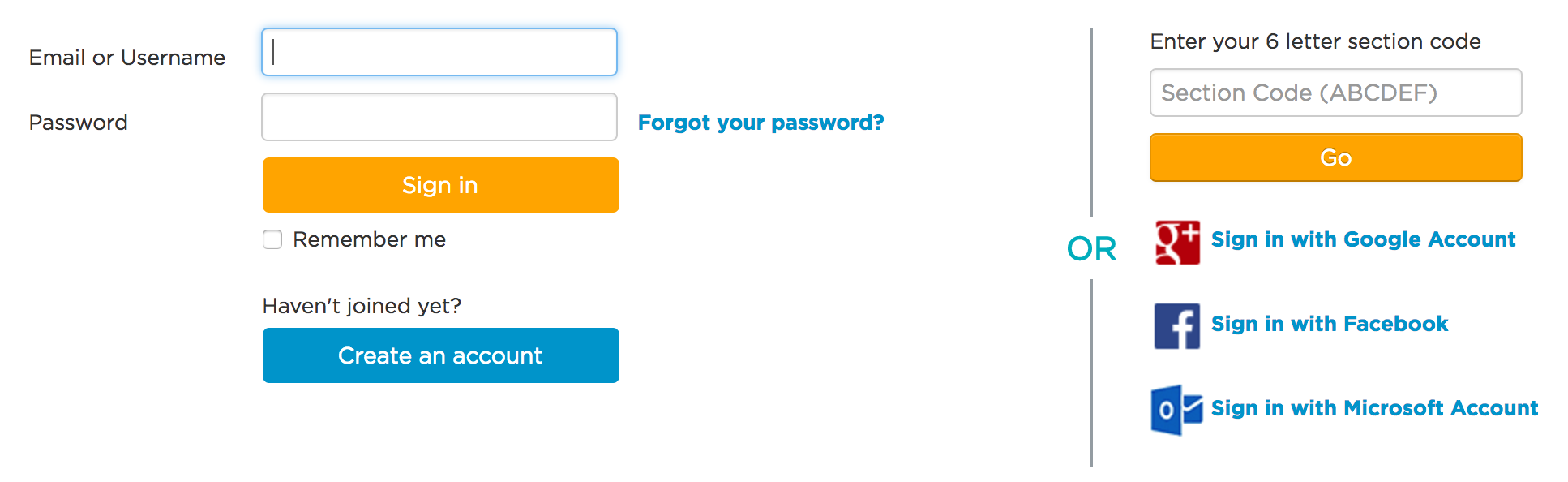The image is a styled user login interface set against a white background, meticulously divided into two sections separated by a thin vertical line. The divider features the letters "O-R" in blue.

On the left section, which occupies approximately two-thirds of the image, there is an entry form for user credentials. At the top, a blue-outlined rectangle is marked "Email or Username" in black text, followed by a similarly styled box below, captioned "Password." Below this area is a clickable text in blue, "Forgot your password?" 

Beneath these fields, an orange rectangle labeled "Sign In" stands out, accompanied by a small check box with the option "Remember me." Further down, blue clickable text reads, "Haven't joined yet? Create an account."

The right section, taking up the remaining one-third, prompts users to "Enter your six-letter section code" with an input box below it. Directly underneath is an orange button with white text that says "Go."

At the bottom, the section has three social sign-in options: a Google Plus icon with "Sign in with Google account," a Facebook icon with "Sign in with Facebook," and a Microsoft logo with "Sign in with Microsoft account."